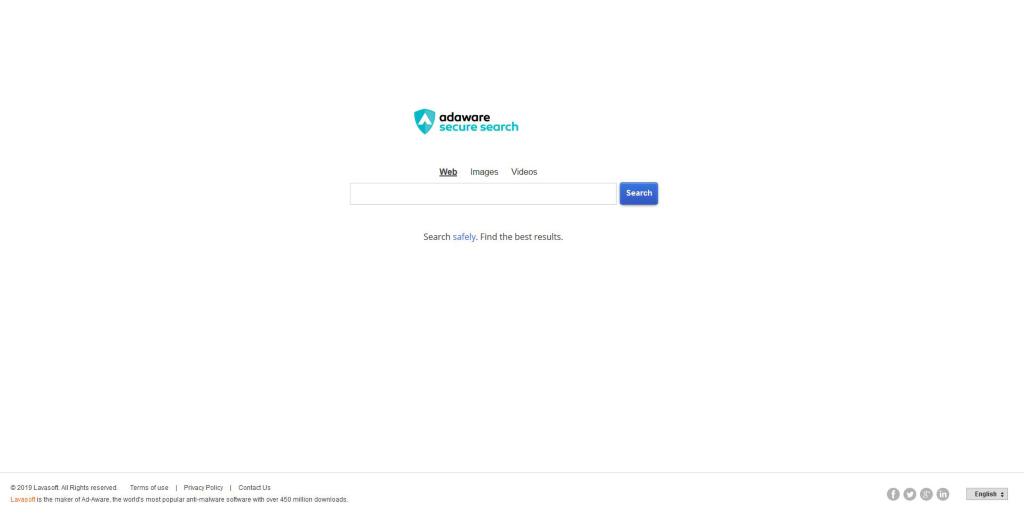**Screenshot of a Simple Search Engine Website Interface**

The website screen features a clean, minimalist design with a white background. 

At the top center of the page is a light blue shield icon, containing a white "A" or an upward-pointing arrow. Positioned beside the shield, the title "AdAware" is prominently displayed in bold black font. Directly below this title, the subtitle "Secure Search" is written in blue font.

Below the header, there are three navigation links: "Web" (currently selected), "Images", and "Videos". Under these links, the main search field is located - a rectangular input area that is currently empty. Adjacent to this field, on the right side, is a blue button with the word "Search" in white font.

A message encouraging safe searches and promising the best results is placed just below the search bar: "Search safely, find the best results."

At the bottom of the page, there is a faint black horizontal line. Below this line, on the right side, are icons for social media platforms including Facebook, Twitter, Instagram, and Google+. Additionally, there is a small gray button labeled "English" in black font.

In the lower left corner, there is a date marker reading "© 2018." Nearby, there seem to be links to legal information like the Terms of Use, though they are not clearly readable.